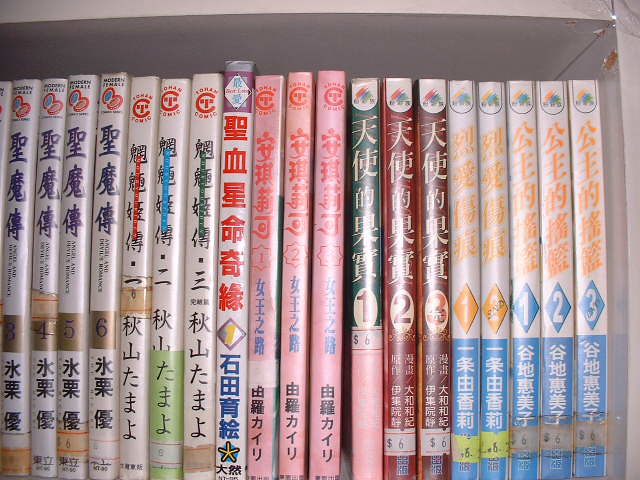The image features a white bookshelf filled with a meticulously arranged collection of books, possibly manga, given the consistent size and format. The books are uniformly aligned, standing upright without tilting, suggesting a well-organized display. They are predominantly in an Asian language, potentially Japanese, given their unreadable characters to the viewer, although a few have small, illegible English text. The collection consists of 17 visible books, with the edge of an 18th book partially in view. These books are grouped in series, indicated by sequential numbering on some of them. The bindings present a vibrant array of colors, including white, pink, red, yellow, light blue, brown, purple, and black. A few books feature price tags marked with $6. Notably, the white bookshelf shows signs of wear; there is noticeable damage on the left side where the paint has chipped, exposing the underlying wood.